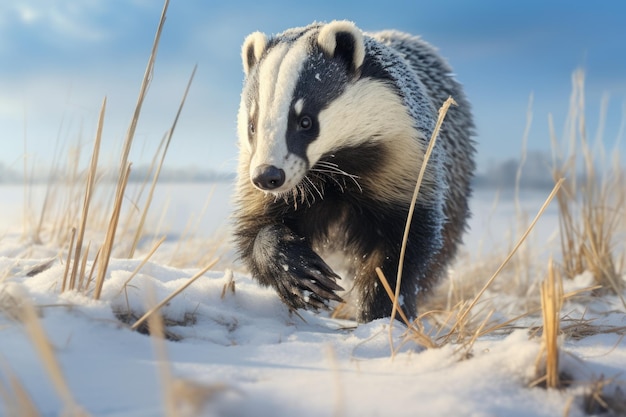This wildlife photograph captures a small, unidentified black and white animal, reminiscent of a skunk or a raccoon, with a longer snout and facial features that might suggest a mink. The scene is set in a snowy, outdoor environment with a clear blue sky and bare trees against the horizon. The snow-covered ground is dotted with beige, dead vegetation protruding through the snow. The animal, with distinctive striped black and off-white or grayish fur, sharp clawed paws, and roundish ears, appears to be walking calmly through the shallow snow. Its fur looks slightly dense and almost feathery, particularly towards the back. The image, possibly taken in the early morning as suggested by the slightly melting snow and bright, sunny conditions, showcases the creature's white whiskers and black nose. In the blurred background, any discernible features blend into muted grays, further emphasizing the serene and wintery atmosphere of the photograph.